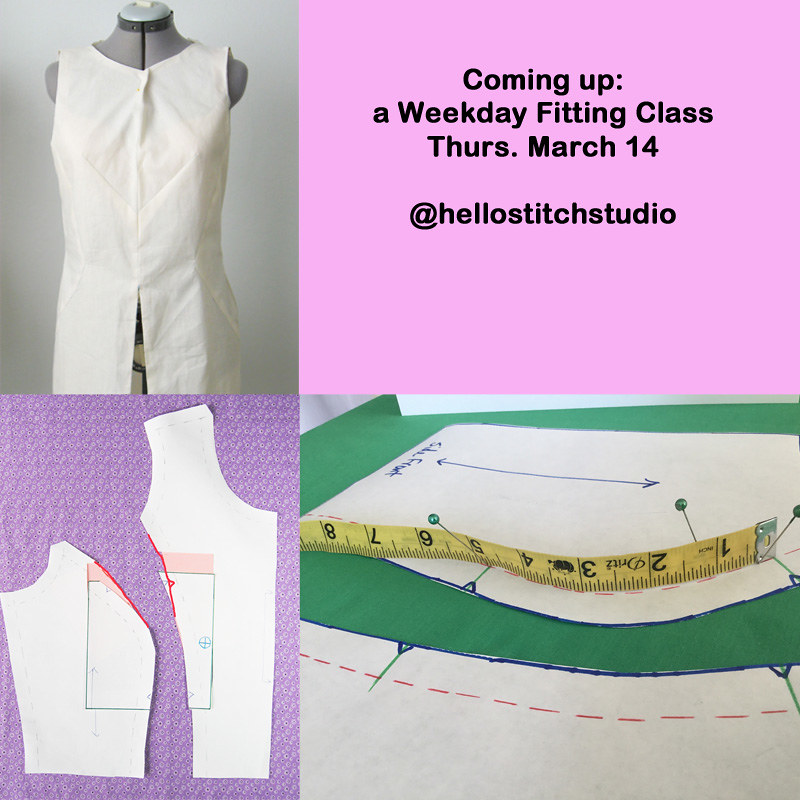The promotional poster is segmented into four distinct sections. In the upper left corner, a headless, armless mannequin stands against a white wall, adorned with a short-sleeved white shirt that is split at the bottom. The upper right section features a lilac purple background with black text that reads, "Coming up: Weekday Fitting Class, Thursday, March 14th at Hello Stitch Studio." The lower left corner displays a dress pattern on dark purple fabric. This pattern, outlined on white paper, includes a blue square and red markings. The bottom right corner offers a close-up view of another dress pattern on green fabric, secured with green pushpins holding a yellow fabric tape measure. Both dress pattern sections showcase red broken dotted lines and blue marker details.